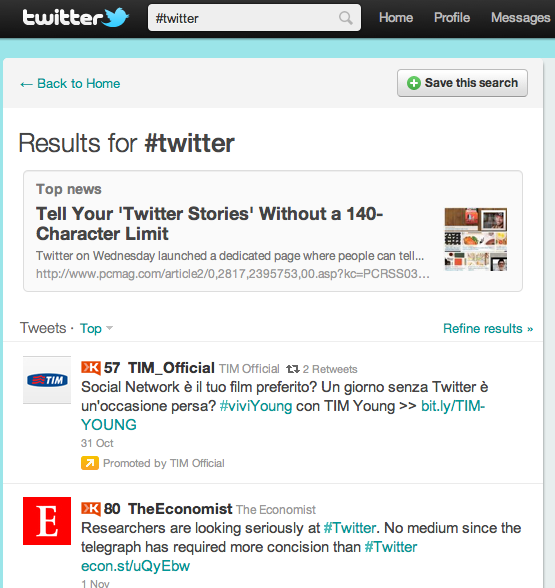This image showcases the search results page of an old Twitter interface, likely from around 10 years ago, exuding a classic design. The top bar is a prominent black strip featuring the iconic Twitter bird logo with 'Twitter' written beside it and a centered search bar displaying '#Twitter.' To the right of the search bar are three gray buttons labeled 'Home,' 'Profile,' and 'Messages.'

Directly below this, the search results are displayed. The upper left corner features a gray bar with blue text and an arrow pointing left, indicating 'Back to Home.' On the right side of this bar, there is a rectangular button with a green circle and a plus icon, reading 'Save this search.' Beneath this, 'Results for #Twitter' is prominently displayed.

Within the results, a gray box titled 'Top News' lists a news summary that reads: "Tell your Twitter stories without a 140 character limit. Twitter on Wednesday launched a dedicated page where people can tell..." This entry includes a URL leading to the full news story and a preview image on the right.

Below the 'Top News' section, there is a smaller 'Tweets' section with the 'Top' label in blue text. The first tweet is from the account TIM_official, written in Spanish: "Social network a you to a feel my preferrito. Un giorno senza Twitter e un ocasion per sa. #ViviYoung con Tim Young," followed by a Bitly link. The next tweet is from The Economist, stating: "Researchers are looking seriously at #Twitter. No medium since the telegraph has acquired more concision than Twitter. #Twitter," with a link to The Economist's website.